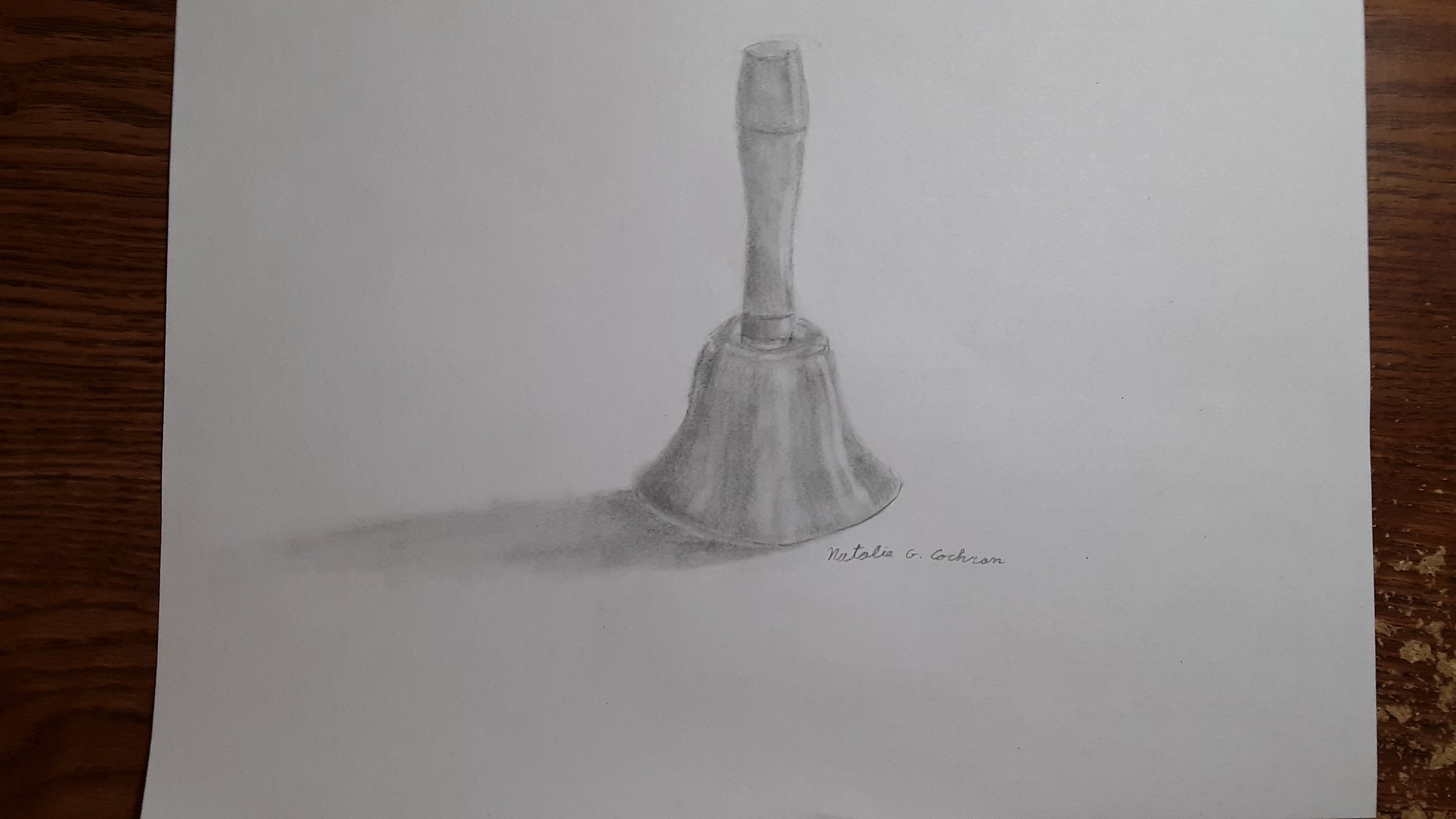The image showcases a detailed black and white pencil sketch of a handbell centered on a white piece of paper. The bell, rendered with fine detail, features a traditional bell shape with a long wooden handle attached via a brass ring. The handle, approximately double the height of the bell, is cylindrical and leads into the bell's body. The artist has skillfully added shadowing to the left of the bell, suggesting a light source from the right. At the bottom right of the paper, the artist's cursive signature reads "Natalie G. Cochran." The paper rests on a dark brown wooden table with a visible grain pattern running horizontally, and a small chip in the wood is notable at the bottom right corner, revealing a lighter brown underneath. The intricate detailing and the monochromatic palette enhance the classic and timeless feel of the artwork.